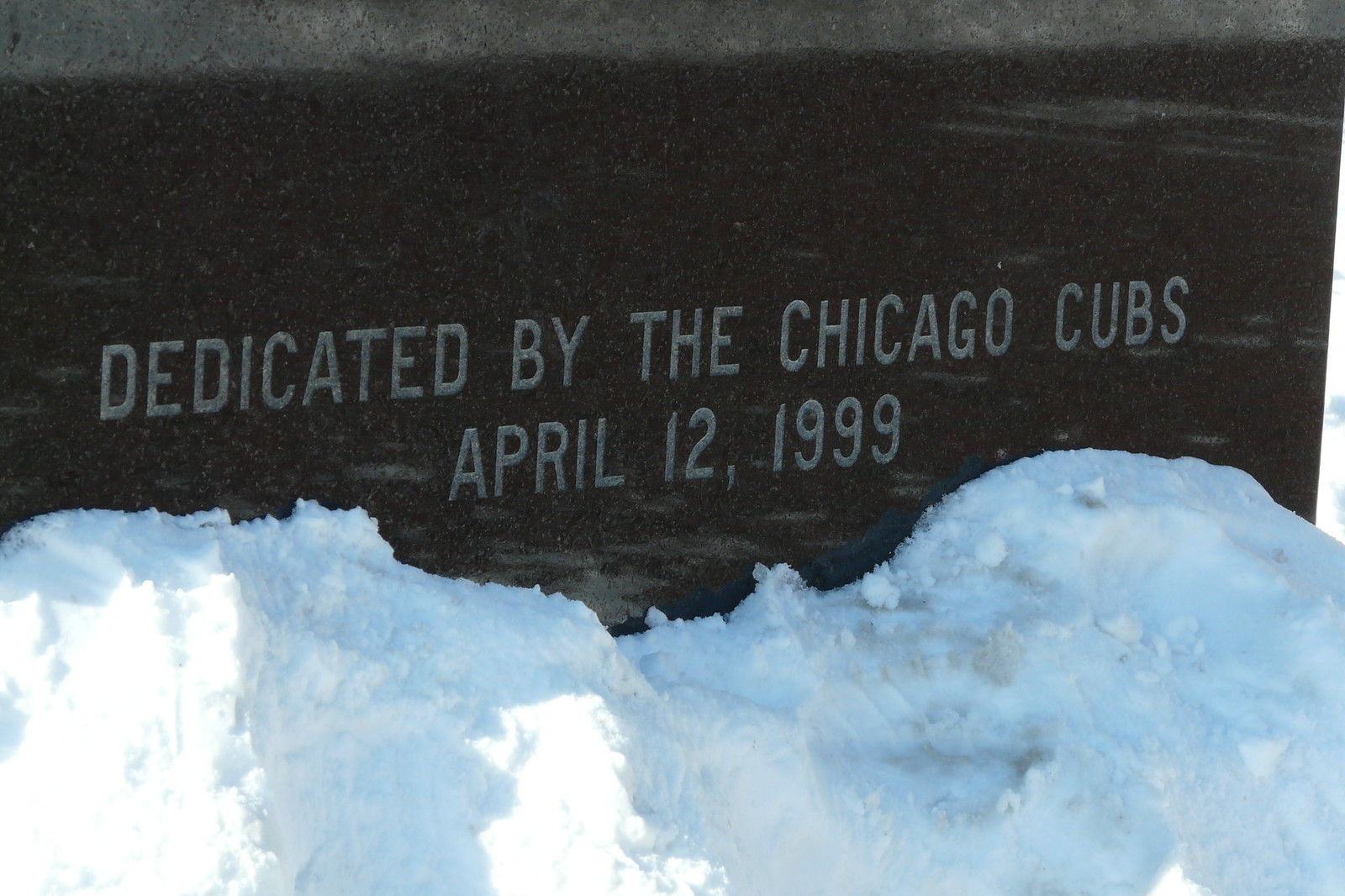This photograph captures a memorial sign, dedicated by the Chicago Cubs on April 12, 1999. The sign, made of a dark or charcoal-colored marble with gray, all-capital engraved letters, occupies the entire background of the image. A slight reflection or glare can be seen on its surface. In the foreground, there is a buildup of snow, forming a drift that is lower in the center and higher on the ends, possibly from being shoveled or piled rather than naturally accumulating. The snow is not high enough to obscure the wording on the sign. The outdoor scene, presumably in Chicago, also shows faint traces of footprints in the snow near the memorial.